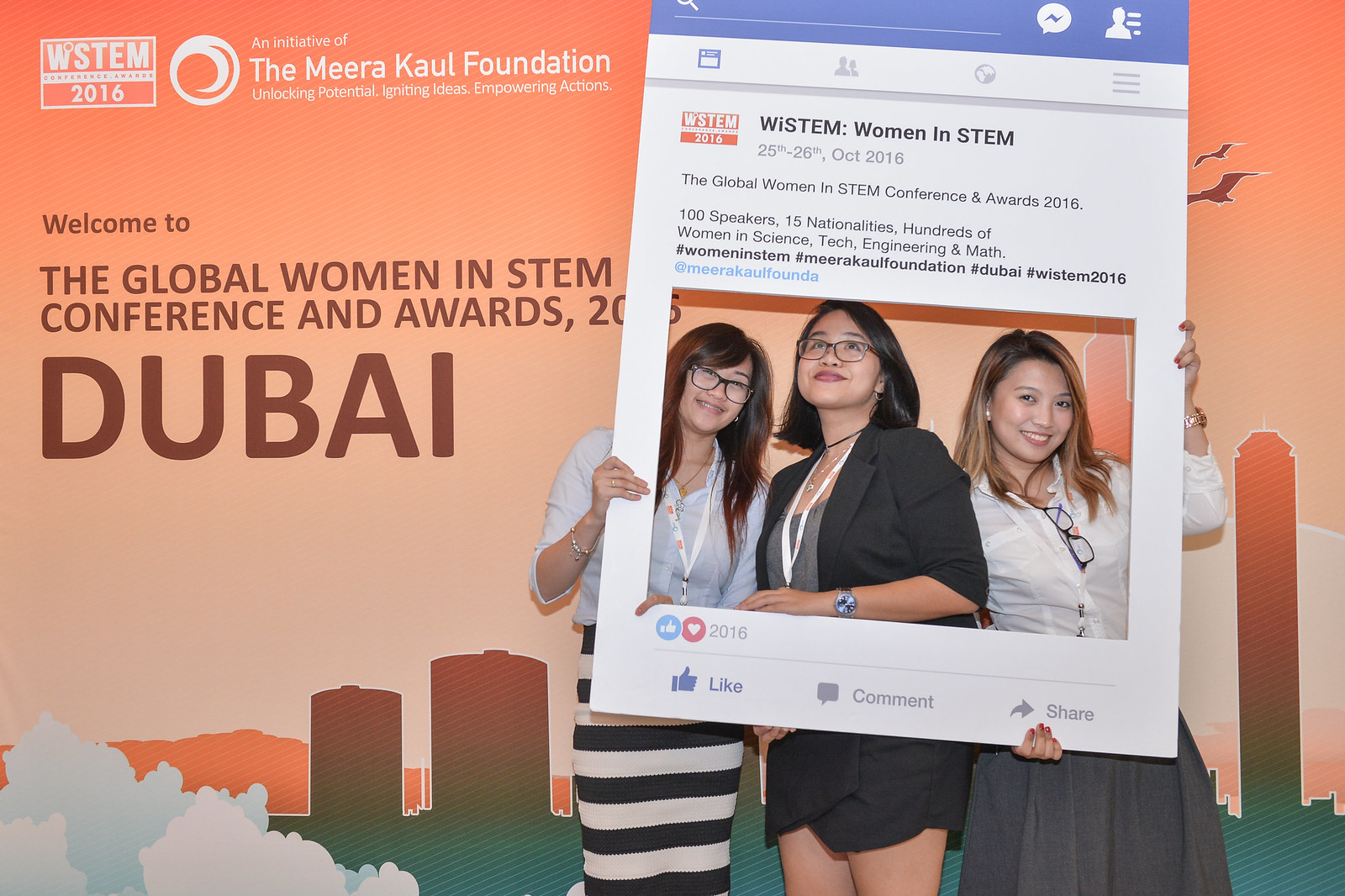The photograph features three young women of Asian descent posing at the Global Women in STEM Conference and Awards held in Dubai in 2016. They are standing behind a large cardboard cutout designed to look like a Facebook page, labeled "Wisdom Women in STEM." This cutout frames their faces as if they are the profile pictures on the webpage, and they are smiling warmly at the camera.

The woman on the left has long hair, wears glasses, a pale blue top, a white lanyard, and a black and white striped long skirt. The central woman, also wearing glasses, has long dark hair, a dark coat over a gray shirt, and a dark skirt with a matching lanyard. The woman on the right has long hair and accessorizes her attire—a white shirt and gray skirt—with glasses hanging from the top button of her shirt, alongside a lanyard around her neck.

Behind them is an orange-salmon colored backdrop with a skyline silhouette of Dubai and text reading "WSTEM 2016, an initiative of the Miracle Foundation" and "Welcome to the Global Women in STEM Conference and Awards, Dubai." The vibrant background and their formal yet stylish attire complement the professional and celebratory spirit of the event.